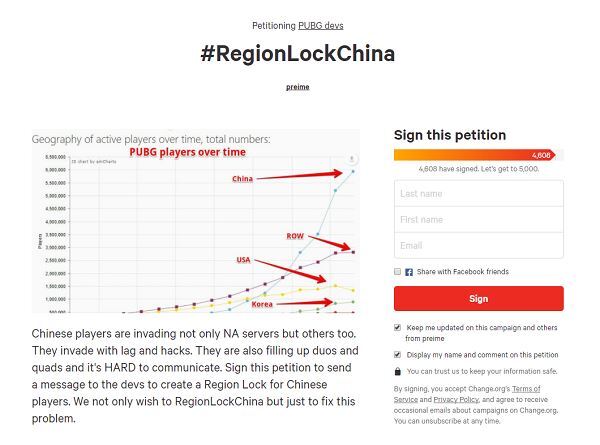The image displays a detailed petition urging the developers of PUBG to implement a region lock for Chinese players, marked by a prominent hashtag #RegionLockChina in bold, black letters. Below, the text reads "Pre-PREIMA," next to a large gray square labeled "Geography of Active Players Over Time - Total Numbers." 

Within the gray square is a graph titled "PUBG Players Over Time" in red, depicting data through three lines: yellow (flat), red (slightly increasing), and blue (drastically rising). The graph is intended to illustrate the influx of Chinese players in various servers, alongside issues of lag, hacks, and communication difficulties in duos and quads matches. 

The petition appeals to players to sign and convey their support for a region lock solution, not just to isolate China, but to address these gaming problems comprehensively. On the right side, there is a sign-up section showing the number of signatures collected, a red sign button, and an option to share the petition with Facebook friends.